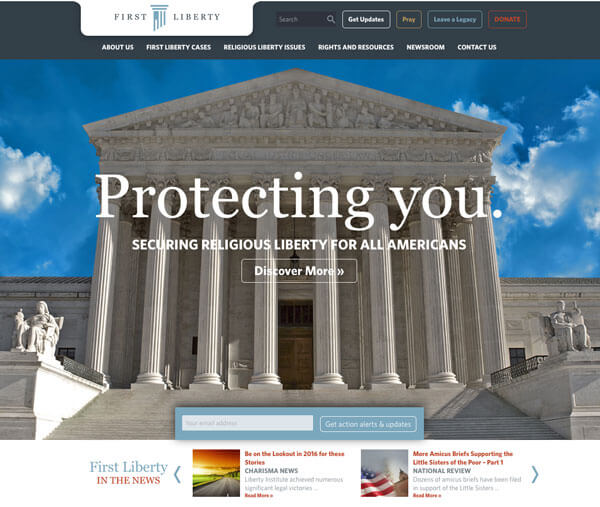**Caption:**

This image, sourced from a website, features a distinct layout with multiple sections. The top inch and a half are adorned with a dark blue border, which includes a small white tab extending downward about two-thirds of the way before curving back up and stretching horizontally about three inches. Inside this tab, there is an emblem resembling an upside-down hanging flag with two or three blue lines above it, accompanied by the word "First." To the right of this, within the same dark blue border, the word "Liberty" is displayed.

Adjacent to this section, there is a darker blue search bar accompanied by a gray-bordered tab that reads "Get Updates" in white text. Further along, a yellow-bordered section displays "PRWI," followed by a light blue-bordered tab that is partially illegible, likely saying "leave" or something similar. Nearby, a red tab with the word "Donate" is prominently visible.

Below this primary navigation bar, on a black background, the text "About Us," "First Liberty Cases," "Religious Liberty Issues," "Rights and Resources," "Newsroom," and "Contact Us" is listed in white. The majority of the image is dominated by a large photograph of a grand stone building featuring eight massive concrete columns, with statues of seated figures at the base of each column on both the left and right sides. The sky above is a vivid blue, dotted with clouds particularly visible mid-left and mid-right within the frame.

At the very bottom of the image, almost touching the edge, there is another blue rectangle housing a secondary search bar. Beneath this, additional news and information sections can be seen, further elaborating on the content of the website.